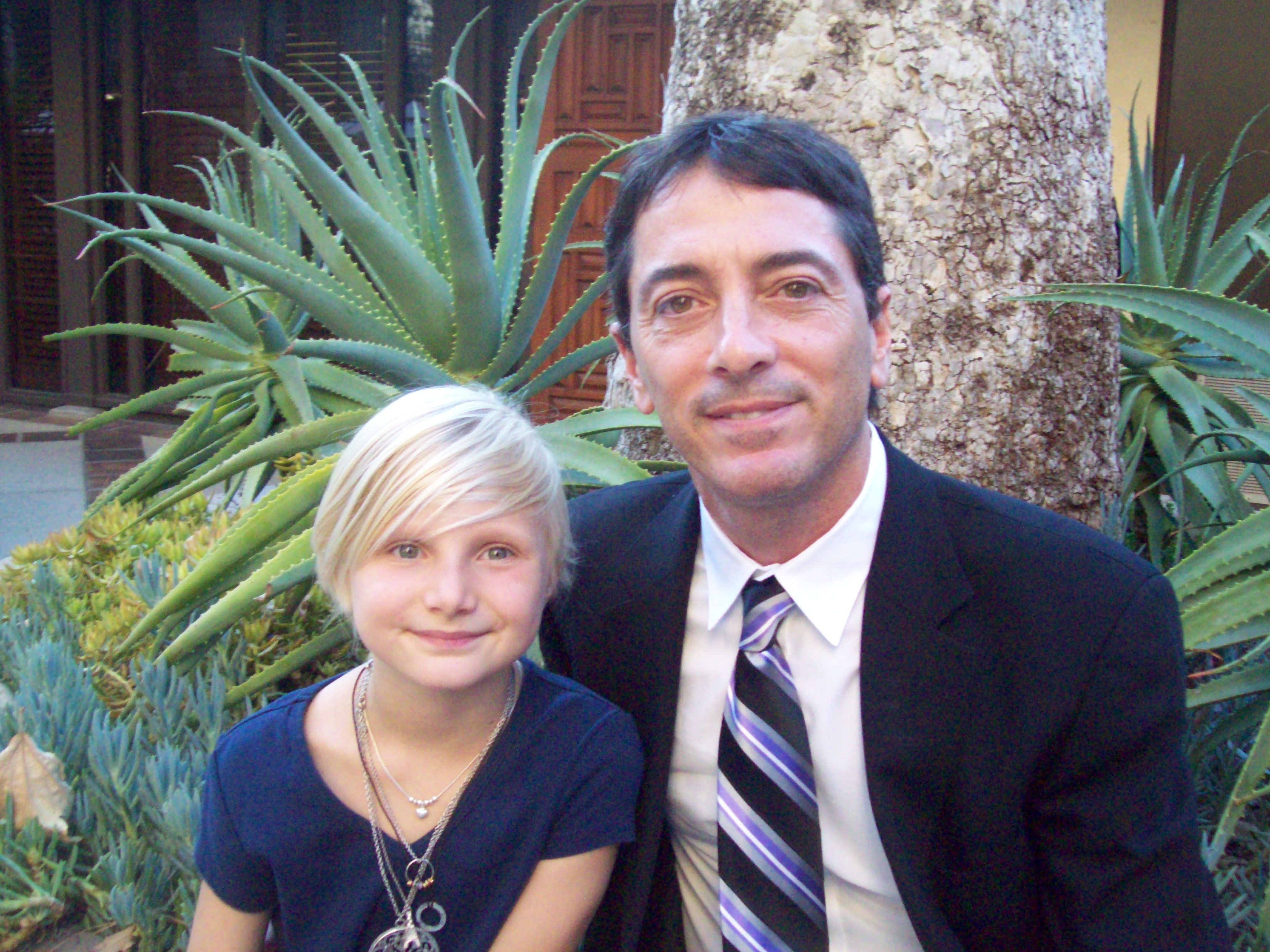This outdoor photograph captures Scott Baio sitting with a young girl who appears to be his daughter. They are positioned on the edge of a raised garden or planter area, with the trunk of a tree and various plants, including aloe or decorative cacti, behind them. Scott Baio, positioned on the right, is dressed for a formal occasion in a dark suit jacket, a white button-down shirt, and a distinctive tie featuring thick black stripes interspersed with a multicolored stripe of lavender, purple, blue, and white. He has short dark hair parted slightly off-center, dark brown eyes, and displays a gentle, intentional half-smile as he faces the camera. Visible wrinkles around his eyes suggest he is likely in his early 40s. Leaning slightly into him is a young girl, markedly shorter by at least a head or head and a half, estimated to be around 8 to 10 years old. She wears a v-neck purple or dark blue t-shirt, adorned with several silver necklaces, some featuring simple pendants and others holding rings. Her light blonde hair sweeps across her face, nearly reaching her eyebrows, and her green-blue eyes mirror Scott's gaze towards the camera. She smiles more naturally, exuding a youthful vibrancy. The background also includes glimpses of a building with windows and possibly a doorway, enhancing the familial and warm atmosphere of the image.